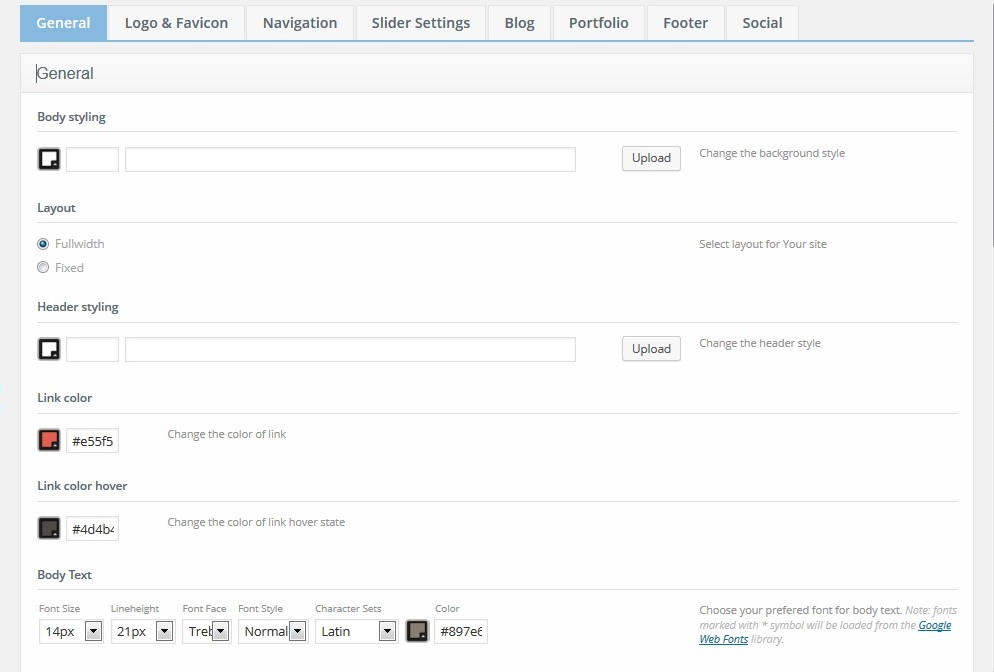Detailed Image Caption:

The image is a screenshot of a settings page designed with a white background enclosed by a gray border. Across the top, a series of tabs are visible, labeled as follows: General, Logo and Favicon, Navigation, Slider Settings, Blog, Portfolio, Footer, and Social. Below this, a thin blue line spans the width of the page, and directly beneath it lies a sizable gray rectangle labeled "General." 

Within the "General" section, various website customization options are displayed. 

The first option is "Body Styling," which includes a prominently bolded label and a text box adjacent to it. Alongside the text box, there is an "Upload" button for changing the background style.

The next option is "Layout," featuring choices for either "Full Width" or "Fixed" configurations. To the right of these choices, descriptive text reads, "Select Layout for your site."

Further down, the "Header Styling" section is presented, comprising a black rectangle with a corresponding text box for uploading and changing the header style.

For "Link Color," the current color is red (#E55F5). The accompanying instruction reads, "Change the Color of the Link."

The "Link Color Hover" option follows, with the hover state color displayed as black (#4D4B). The prompt beside it says, "Change the Color of the Hover State."

The final setting within this section is "Body Text," which has detailed typography specifications: a font size of 14 pixels, line height of 21 pixels, the font face "TREB," normal font size, character sets for Latin, and a font color specified as #897EF.